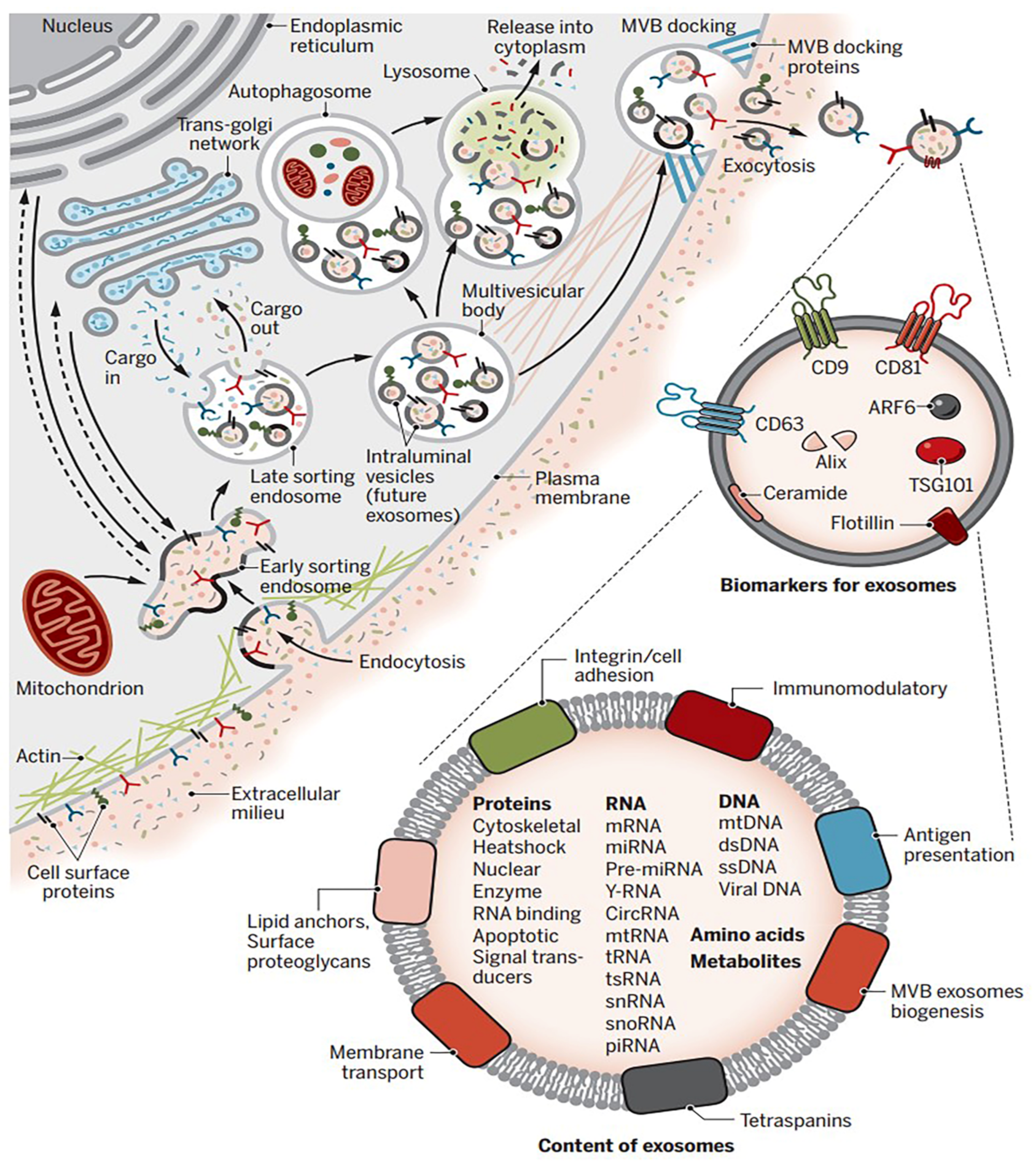This highly detailed scientific illustration, resembling a page from a medical textbook, portrays a human cell with a focus on exosomes. The top left corner of the image features a gray-blue background and a black-labeled nucleus, along with concentric ovals outlined in white and gray. The main body of the diagram is populated with circles and ovals interspersed with red and green dots. To the bottom right, there's a circular structure listing various proteins, including cytoskeletal, heat shock, nuclear, enzymes, RNA-binding, and apoptotic signal transducers. The RNA category enumerates different types such as mRNA, miRNA, pre-miRNA, yRNA, circRNA, mtRNA, tRNA, tsRNA, snRNA, snoRNA, and piRNA. The DNA section lists mtDNA, dsDNA, ssDNA, viral DNA, along with amino acids and metabolites.

This image also intricately illustrates cellular processes and structures such as endocytosis, plasma membranes, exocytosis, extracellular milieu, and cell surface proteins. In addition to portraying endoplasmic reticulum and mitochondrion, it includes detailed depictions of integrin solidation, antigen presentation, and membrane support. Labels identify various features related to cellular function, highlighting the complex interactions within the cell. This elaborate diagram aims to elucidate how these processes and components interrelate, making it an essential visual aid for understanding the multifaceted functions of cellular biology.